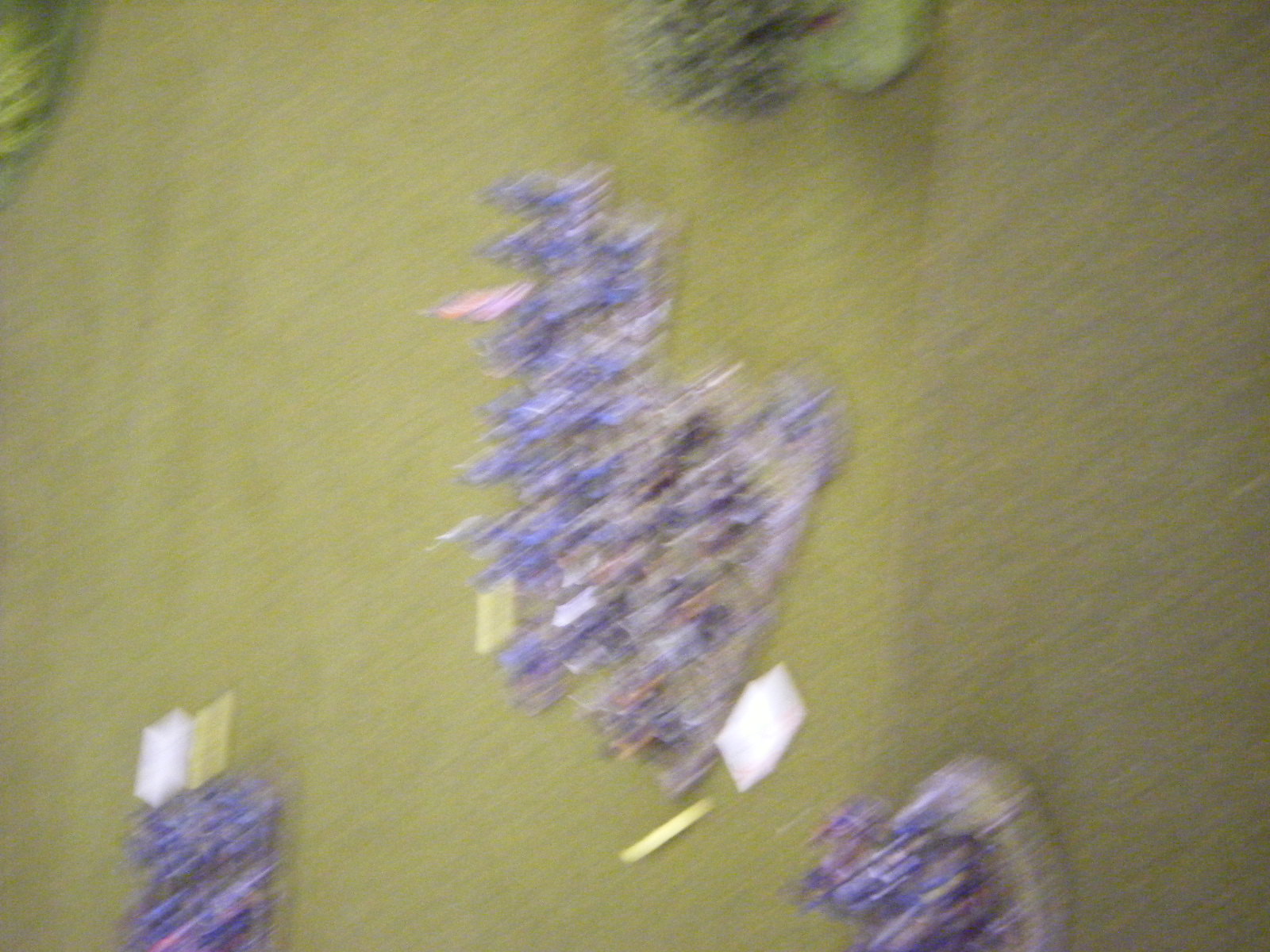In this out-of-focus image, a colorful scene unfolds against a backdrop of green felt. Central to the image are vibrant purple elements, potentially flowers or crystals, accentuated with hints of white at the tips. The bottom-left corner features a yellow sticky note, contrasting with a piece of white paper lying next to it toward the bottom right, accompanied by what seems to be a yellow stick. The top right displays a cluster resembling a head of broccoli, adding a lush, green plant-like detail. Meanwhile, the top left showcases a dark green object adorned with alternating dark and light green stripes, contributing to the overall textured and vibrant composition.